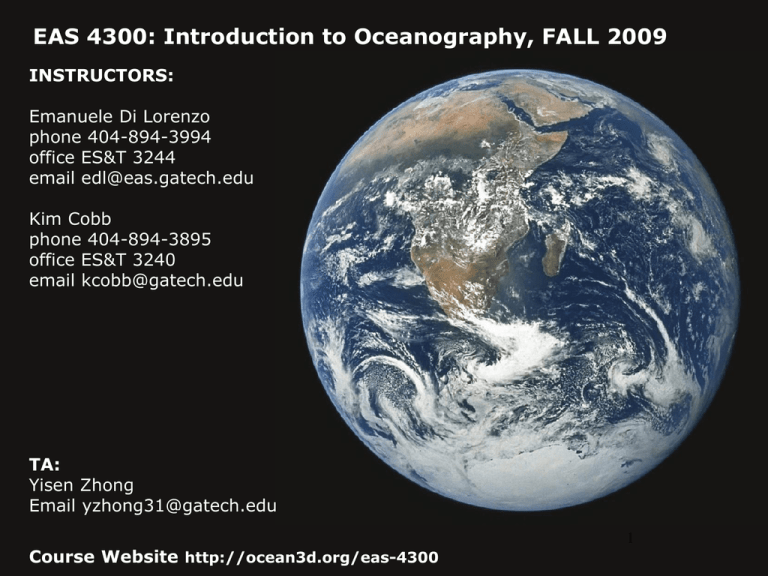This image is a detailed introductory slide for a course titled "EAS 4300: Introduction to Oceanography, Fall 2009." The background is black, with a prominent visual of Earth from outer space situated on the right side, taking up a significant portion of the image.

In the top left corner, the course title is presented in bold, white, all-uppercase letters. Below the course title, the word "INSTRUCTORS" is also capitalized, indicating the section dedicated to instructor information. 

The information for the first instructor is as follows:
- Name: Emmanuelle D. Lorenzo
  - Phone: 404-894-3994
  - Office: ES&T 3244
  - Email: edl@EAS.GATECH.edu

A blank line separates the information for the second instructor:
- Name: Kim Cobb
  - Phone: 404-894-3895
  - Office: ES&T 3240
  - Email: kcobb@GATECH.edu

Following another space, the details for the teaching assistant (TA) are displayed:
- Name: Yesen Zhong
  - Email: YZHONG31@GATECH.edu

At the very bottom of the image, the course website is mentioned, but the exact web address is not specified in the provided description.

Overall, the slide efficiently conveys all essential contact information for the EAS 4300 course instructors and TA, set against a visually striking image of Earth from space, emphasizing the theme of oceanography.